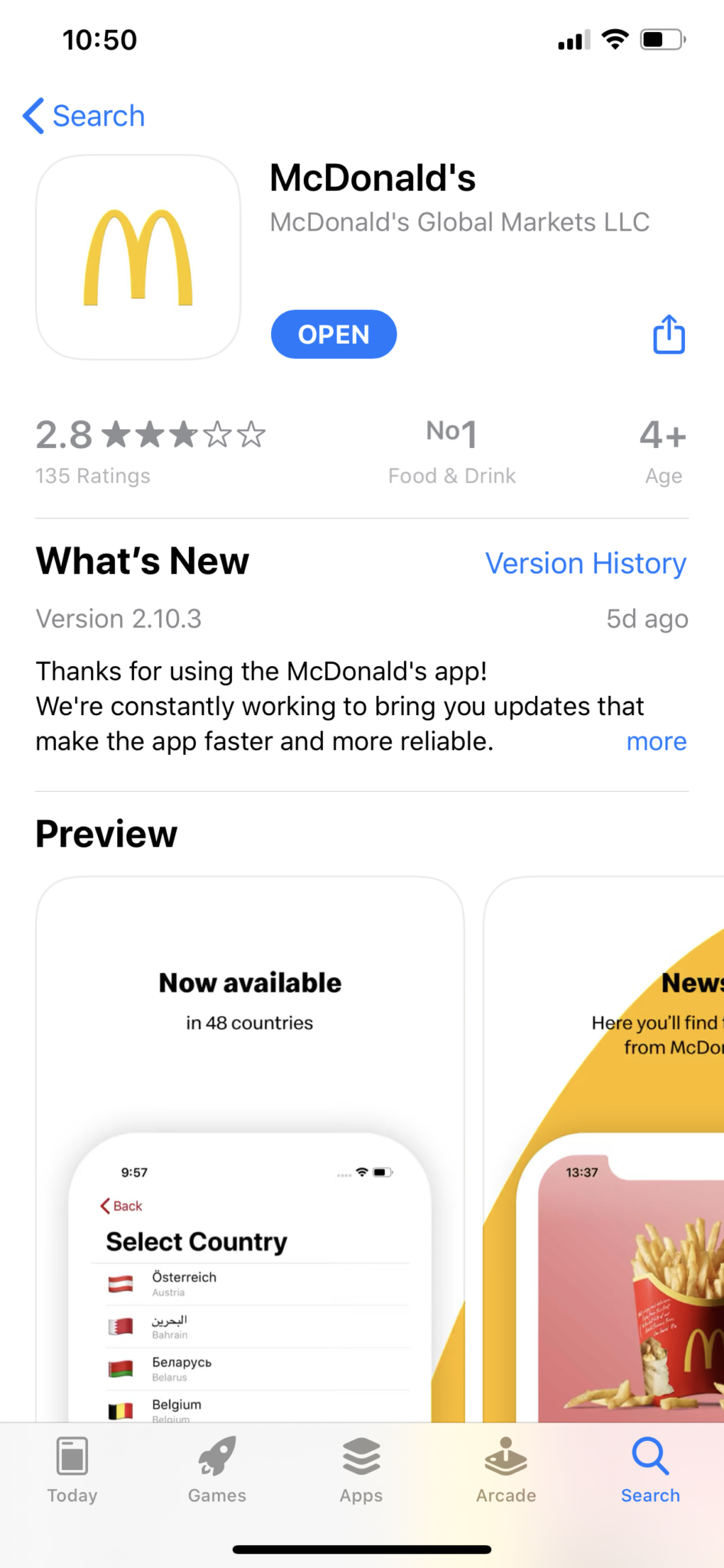This screenshot, taken from an iPhone, captures the McDonald's app displayed in the iOS App Store. In the upper-left corner of the screen, the time reads 10:50, although it doesn't specify whether it's a.m. or p.m. On the upper right, we see connectivity indicators showing a strong cellular signal with four out of five bars and full Wi-Fi strength with three bars. The battery icon reveals approximately 40-50% charge remaining.

At the top center of the screenshot, the text reads "McDonald's App," directly underneath which "McDonald's Global Markets LLC" appears, identifying the developer. The iconic McDonald's logo is prominently displayed to the left of this text. Above this, further to the left, the word "Search" appears in blue, accompanied by a blue arrow, indicating the option to return to the previous screen. A blue "Open" button is also visible, signifying that the McDonald's app is already downloaded and installed on the device. This button provides a shortcut to launch the app directly from the App Store interface.